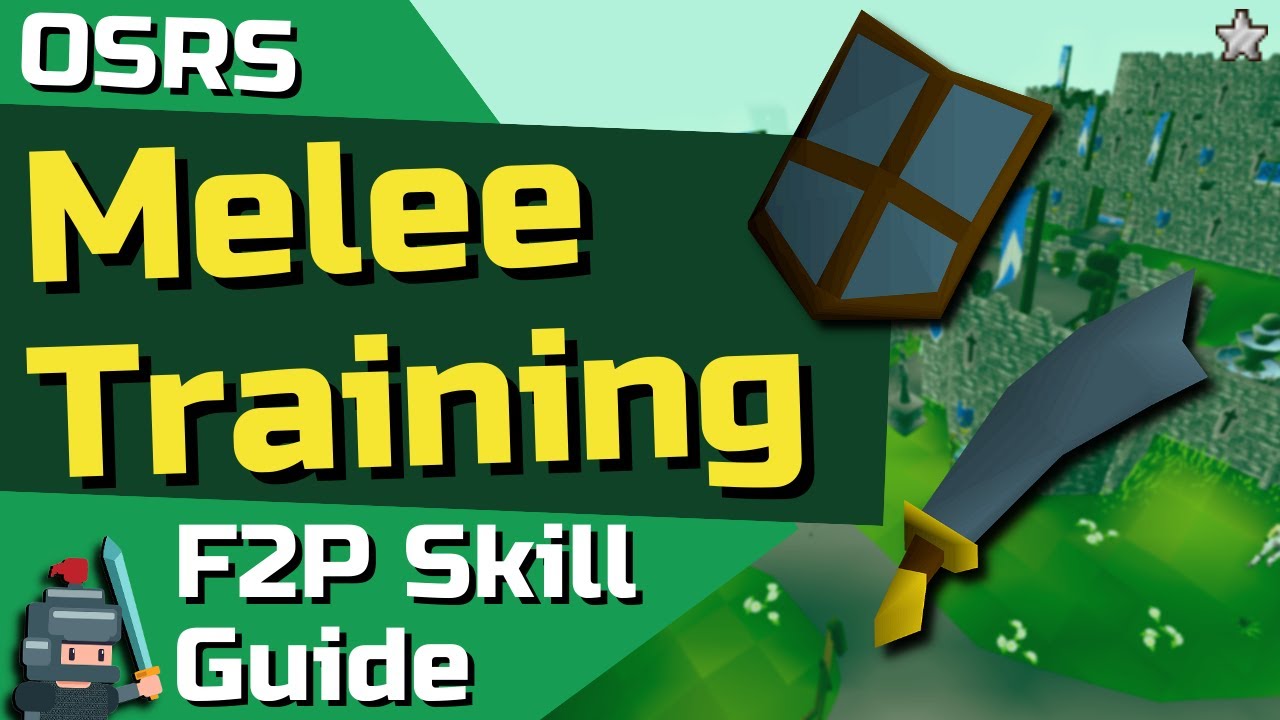The image is a detailed, green and brown social media advertisement for a skill guide for Minecraft, designed in a digital style reminiscent of video games. Dominating the background is a Minecraft-themed game scene, accentuated by various objects from video games. On the left, in prominent white letters, it reads "OSRS." Below, in big yellow letters within a green rectangular box, it says "Melee Training." Further down in white letters, "F2P Skill Guide" is displayed. The bottom left showcases a Minecraft-shaped character, resembling a knight, wearing gray armor with a red tassel atop the helmet and holding a raised sword. On the right, the image features additional game elements: a rudimentary cartoon-style green castle with a silver star, a prominent gray sword with a yellow handle, and a medieval-style gray shield outlined in brown wood with a brown cross in the center.